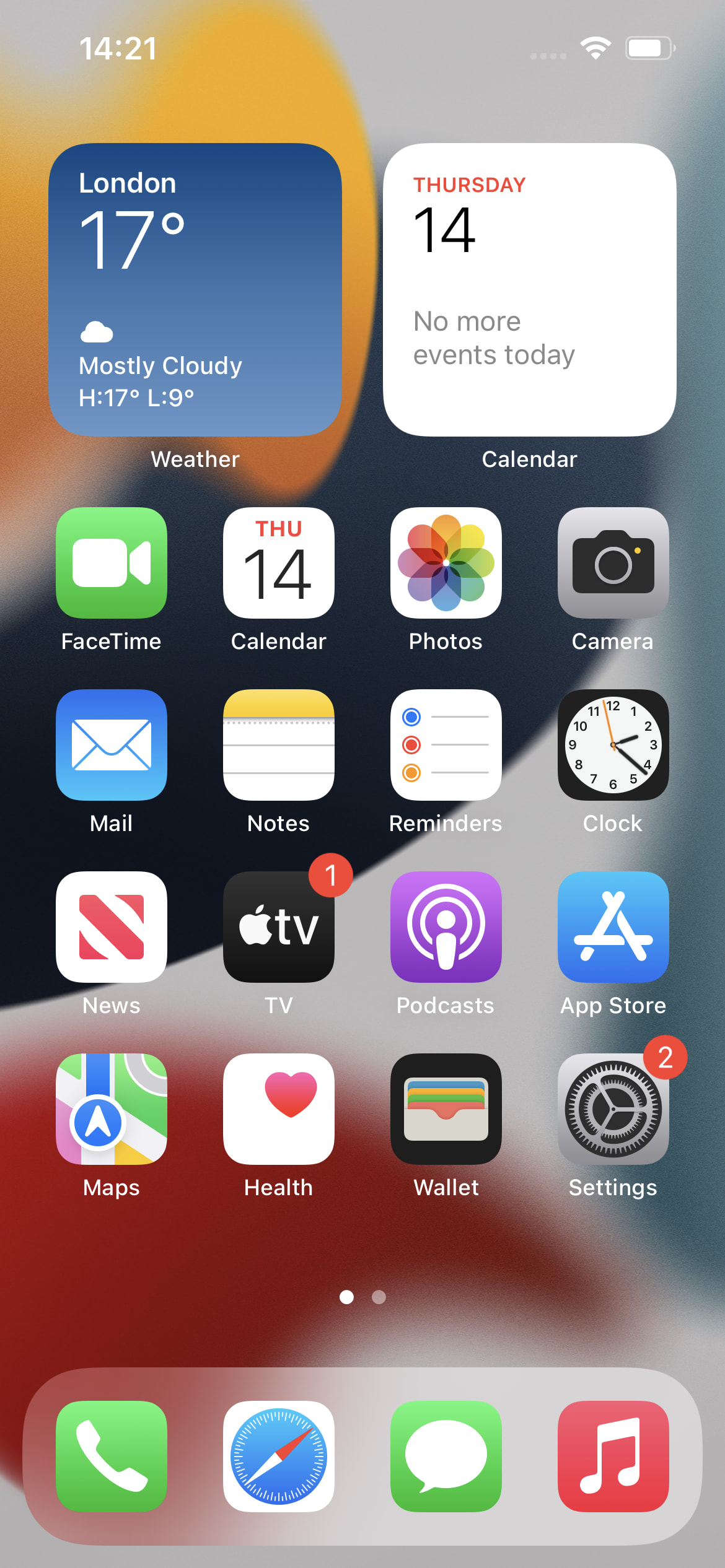The image is a neatly arranged screenshot of an iPhone's homepage, prominently featuring two widgets at the top. 

- **Top Left Widget: Weather**
  - Shape: Square with rounded edges
  - Information Displayed: 
    - Location: London
    - Temperature: 17 degrees
    - Weather Icon: Cloudy
    - Description: Mostly Cloudy
    - Temperature Range: High 17 degrees, Low 9 degrees (abbreviated as H 17°, L 9°)
    - Label: Weather
  - Color Scheme: White text on a muted, artistic background transitioning from yellow at the top to black and white below, creating a blurred effect.

- **Top Right Widget: Calendar**
  - Background: White
  - Header: Red text reading "Thursday"
  - Date: Large black number "14"
  - Additional Info: Text stating "No more events today"
  - Label: Calendar

**Below the Top Widgets: Standard App Grid in Rows of Four**
1. **First Row**: 
   - FaceTime
   - Calendar
   - Photos
   - Camera
2. **Second Row**: 
   - Mail
   - Notes
   - Reminders
   - Clock
3. **Third Row**: 
   - News
   - TV (with a red notification badge)
   - Podcasts
   - App Store
4. **Fourth Row**: 
   - Maps
   - Health
   - Wallet
   - Settings (with two notifications)

**Bottom Dock Bar: Frequently Used Apps**
- Phone
- Safari
- iMessage
- Music

The overall layout is clean, user-friendly, and characteristic of a well-organized iPhone interface.